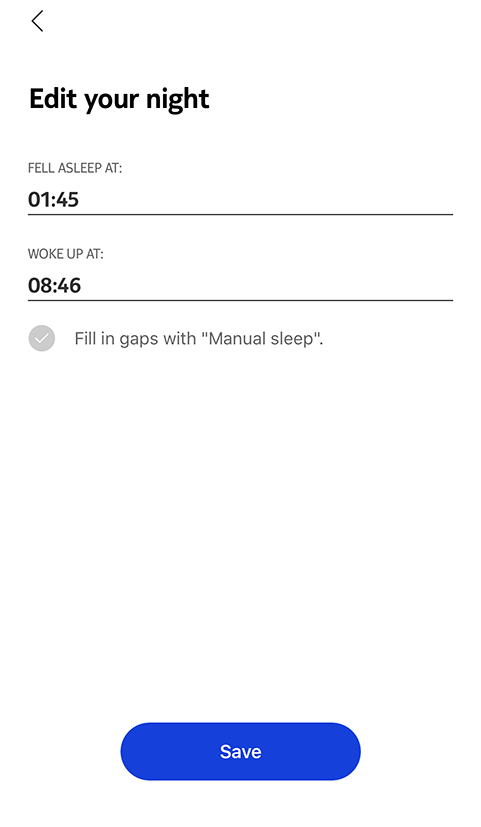The screen of the sleep tracking app displays a minimalist design on a white background. At the top left corner, there's a left-pointing arrow indicating the option to go back to the previous screen. Below the arrow, left-aligned in bold black font, the text reads "Edit Your Night." 

A section follows in smaller, non-bold black font, stating "Fell asleep at:" with the time "01:45" in bold and underlined in black, extending horizontally across the screen. 

Subsequently, there's another section labeled "Woke up at" in the same smaller, non-bold black font, followed by the time "08:46" in bold and also underlined. 

Towards the bottom of the screen, there is a row starting with a gray circle containing a white checkmark, accompanied by the text "Fill in gaps with 'Manual Sleep.'" 

At the very bottom, a prominent blue "Save" button is present, ready for the user to finalize their edits.